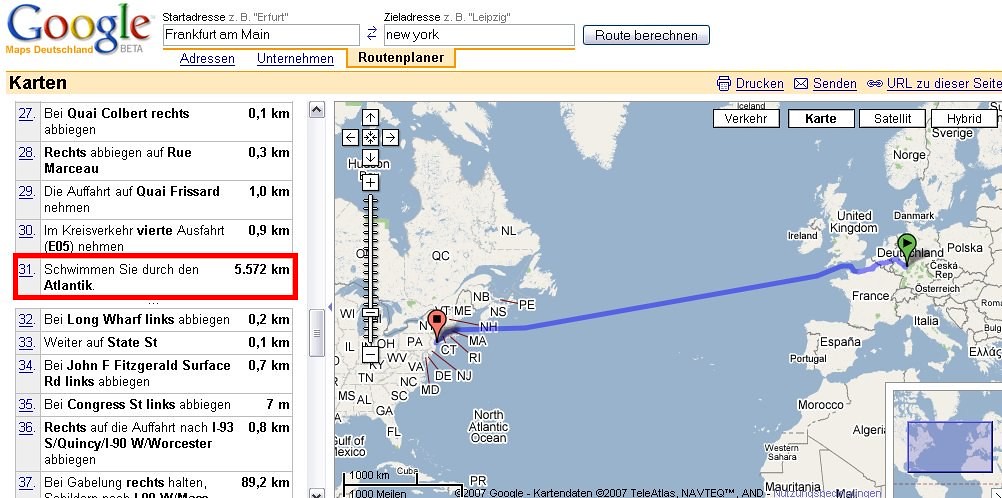The image is an old-style Google Maps interface written in German, displaying a route planner prominently labeled "ROUTENPLANNER" and showing the distance of 5,572 kilometers. The map indicates a route with a dark blue line extending from a red marker near New York City, USA, across the Atlantic Ocean to a green marker in Frankfurt, Germany. The left side of the image lists the directions in German, while the right side features a map encompassing parts of North America, Europe, and Africa, including visible regions like the United States, Canada, Poland (Polska), and a bit of Morocco. At the top, a tan bar runs horizontally with the label "CARTEN" in black letters. The overall interface suggests it's a beta version of Google Maps from an earlier time.